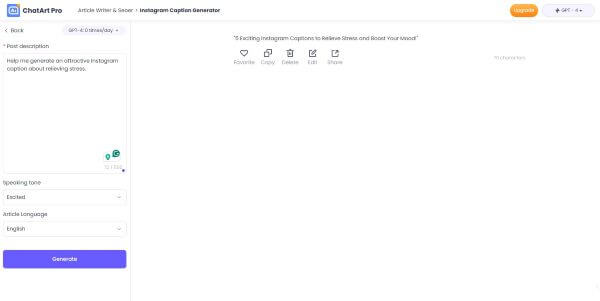This is an image of a webpage titled "Chat Art Pro." In the upper left corner, there is a square icon featuring a central circle with additional details that are not clearly visible. The "Chat Art Pro" text is bolded, though the overall resolution of the image is low, making finer details difficult to discern. Adjacent to "Chat Art Pro," there appears to be faint gray text that says "article," followed by more pronounced bold text which might read "Instagram."

On the right side of the header, there is a button labeled "Upgrade," and nearby, a faded green button is visible. Also on the right, a chat window is present. Above this window, the word "rock" is displayed, alongside a left-pointing arrow and additional, less distinguishable text to the right.

Below this, a section labeled "Description" is enclosed in a small rectangular box. The main content area contains text, with a couple of symbols and numbers located at the bottom right of this section. Additionally, there are two rectangular drop-down boxes positioned below. A prominent long blue button is also visible near the bottom of the webpage.